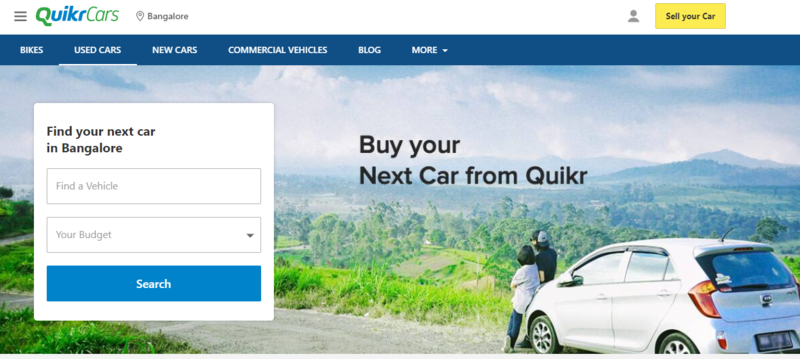The image depicts an advertisement for Quicker Cars, prominently featuring various elements and a scenic backdrop. 

In the upper left-hand corner, the Quicker Cars logo is displayed. On the opposite side, in the upper right corner, there's an icon of a person and a rectangular button labeled "Sell Your Car." 

Beneath these elements, a dark blue banner spans the width of the page. The text on the banner, although somewhat blurry, reads in capital white letters: "BIKES," "USED CARS" (underlined), "NEW CARS," "COMMERCIAL VEHICLES," "BLOG," and "MORE" with a pull-down arrow beside it.

The central portion of the page is dominated by a scenic outdoor photograph. It captures a rural setting with a winding road leading to a white vehicle situated in the lower right corner. Two individuals are seen leaning against the hood of the car, gazing at the picturesque landscape. The background features a heavily forested area with tall mountains and clouds completing the serene view.

Overlaying the middle of the picture, text in bold capital letters reads, "Buy Your Next Car from Quicker." On the far left of the image, a large white square partially covers the scenery. At the top of this square, it states, "Find Your Next Car in Bangalore." Below this is a rectangular text box with the label "Find a Vehicle." Further down, another rectangular box labeled "Your Budget" includes a pull-down arrow. Finally, at the bottom, a blue rectangle with the word "Search" invites user interaction.